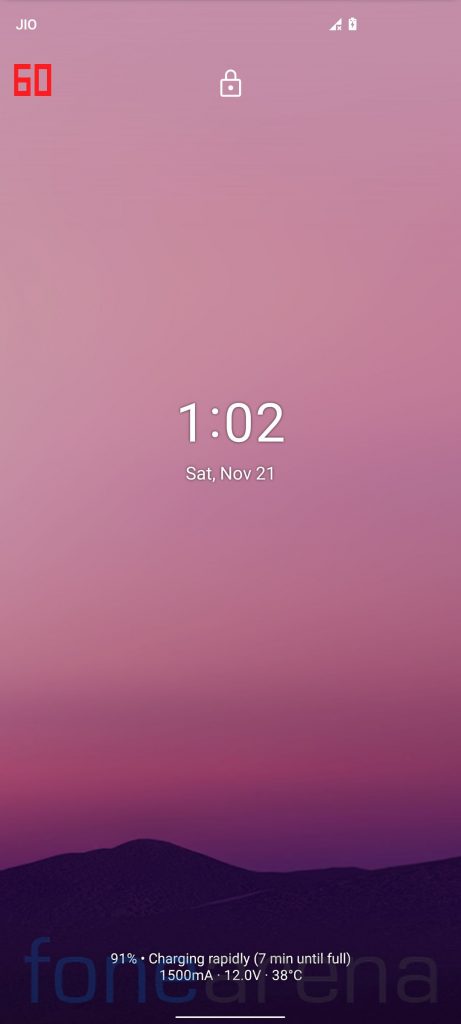The image showcases a cell phone with a visually striking screensaver. The lower portion of the screen features dark brown mountains, while the sky above them transitions through several hues: starting with dark purple just above the mountains, then moving to vibrant hot pink and light purple, and finally blending into a lighter pink towards the top of the screen. 

In the status bar at the top, there are a few icons. On the left side, "JIQ" along with a red "60" is visible. Centrally positioned at the top is a white lock icon, and beneath it, the text reads "1:02", "Saturday," "November 21st." 

At the bottom of the screen, just above the mountains, there is the "Phone Arena" logo where "FONE" is blue and "arena" is in a light gray color. Immediately below this, the charging status is displayed: "91% charging rapidly," indicating "7 minutes until full," along with additional details "1500mA," "12V," and "38 degrees Celsius."